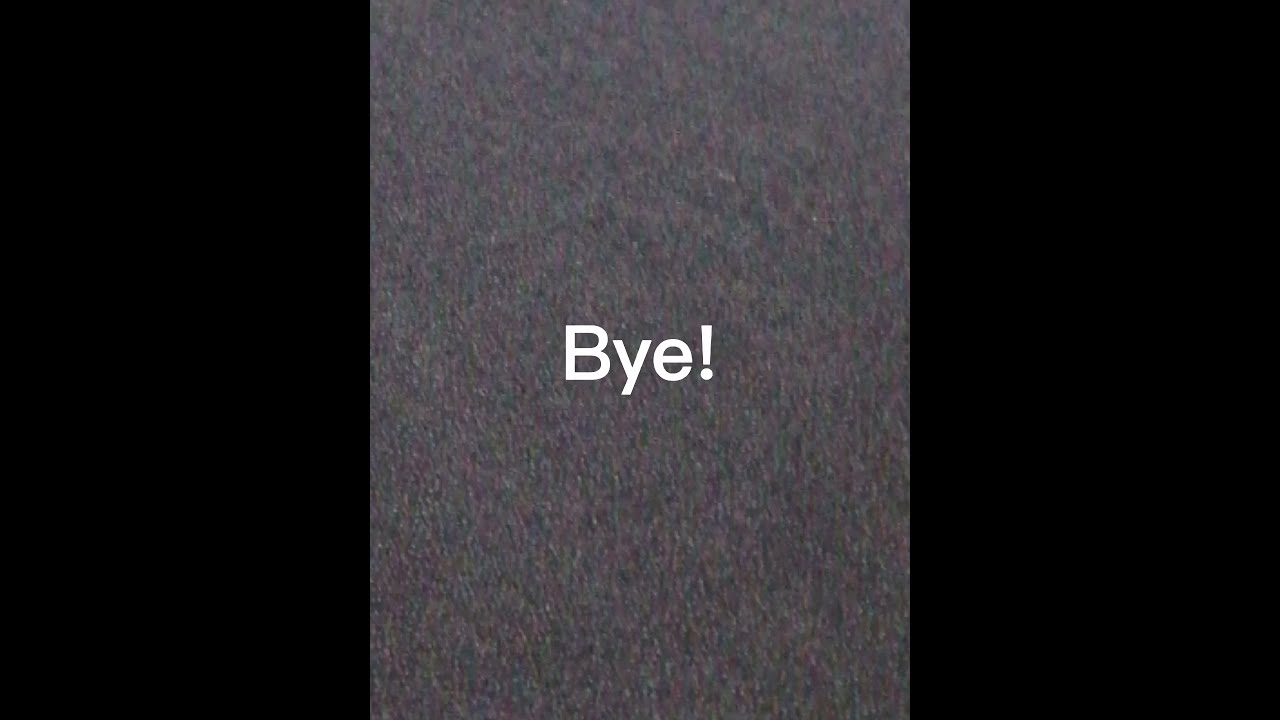This image features a notable rectangular structure with two distinct sections: the outer edges and the central area. The left and right sides of the picture, each taking up slightly more than a fourth of the image, are filled with a solid black background. The central portion, which occupies a little more than a third of the frame, is a textured gray section with a mottled appearance. This gray area contains subtle twinges of various colors, including red, blue, green, yellow, pink, and near-black spots, reminiscent of static on an old television. 

Prominently displayed in the very center of the gray section is the word "by" in white block letters. The 'B' is capitalized, while the 'y' and 'e' are in lowercase, followed by an exclamation point also in white block letters. This text is precisely centered within the gray section, with the background visible through the gaps in the letters and punctuation. The image overall lacks any figures or additional elements, emphasizing the stark contrast and simplicity of its design.